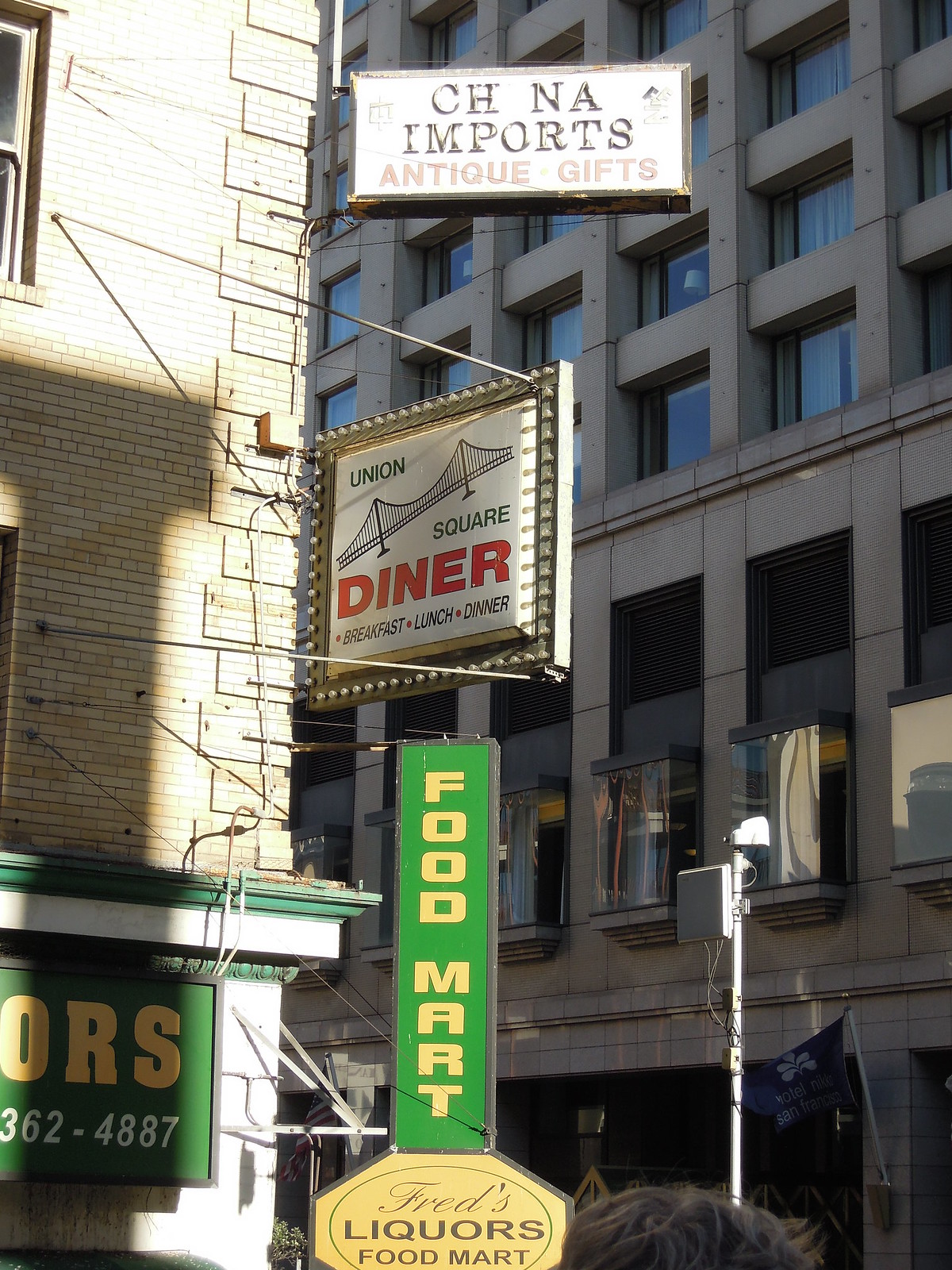The image captures a vibrant street corner scene in a city, possibly Chicago, distinguished by a series of eclectic signs affixed to the corner of a light stone brick building. At the top, a rectangular sign with a gold frame reads "China Imports Antique Gifts," featuring a white background with black and red text, mounted on a metal bracket. Directly below, another sign for "Union Square Diner" stands out with its gold frame adorned with unlit light bulbs; it includes a white background, a clipart illustration of a bridge, and red lettering for "Diner," along with "Breakfast, Lunch, Dinner" in black font. Below this, a tall, green, vertically-oriented rectangular sign states "Food Mart" in yellow font. The next sign, shaped like a hexagon, reads "Fred's Liquors Food Mart" with "Fred's" in cursive and the remaining text in a sans serif font, enclosed by a black circle outline. The building's corner is contrasted by a brutalist-style gray building in the background across the street. Additionally, the top part of a head with dark hair is visible at the bottom of the image, indicating human presence in this urban milieu. The scene is set during the daytime, as evidenced by the natural light and unlit bulbs. No sky is visible, focusing the viewer’s attention on the urban architecture and signage.